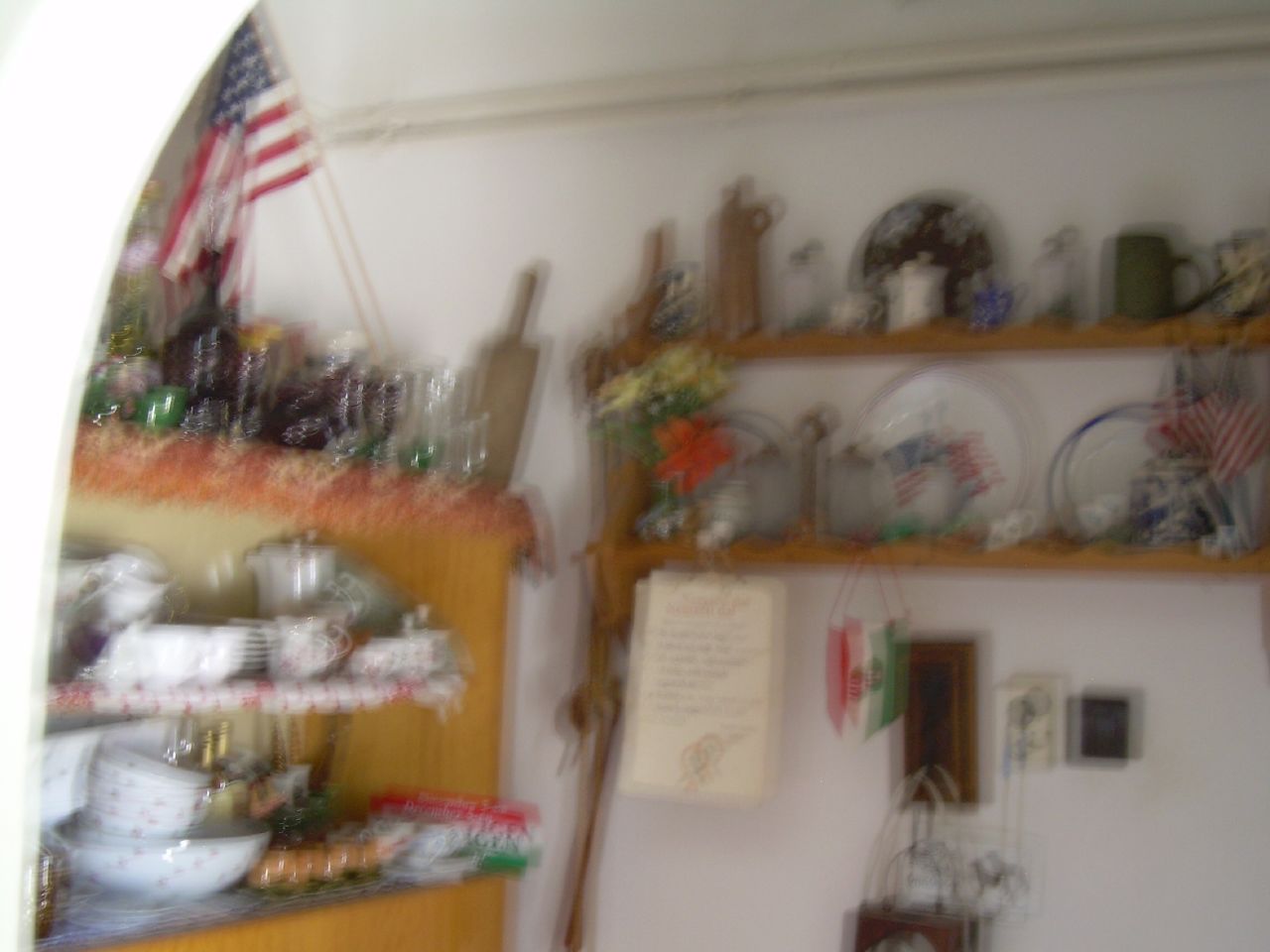The indoor photograph captures a display of ceramics and flag-themed decorations. In the top left corner, there is an American flag, although it is quite out of focus. The setup appears to be an exhibition showcasing American ceramics. On the left side of the image, various bottles, possibly made of metal or glass, are seen in shades of blue and green.

Adjacent to these bottles, there is a wooden shelf holding an assortment of white dishes and framed pictures, all set against a wooden background. The middle section of the photograph features items in white and red hues. At the bottom, a stack of ceramic dishes with delicate floral patterns can be observed.

An array of flags adds an international touch to the display. There is an object with the colors of the Italian flag displayed (red, white, and green), and a flag with the same color scheme but arranged in a manner similar to the Mexican flag. A plate near this area also bears the American flag.

The top part of the image shows a blue dish adorned with white flowers, set against a white wall. Additionally, the brown shelving and a somewhat visible but unreadable posted letter add to the rustic charm of this intriguing and eclectic display.